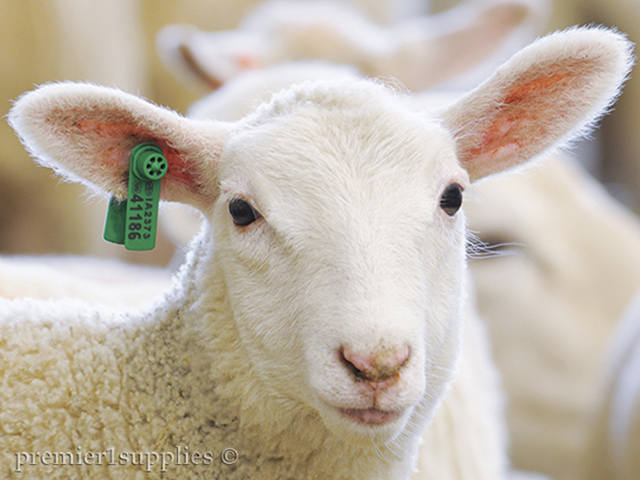The high-definition photo captures a close-up of a white sheep with freshly shorn wool, revealing a clean, pure white face. It is facing slightly to the right, but its head is turned towards the camera, highlighting its pink ears illuminated by the light. The sheep's left ear features a green tag with black text that reads "IA 2373" on the top line and "41186" on the bottom line, with "Premier One Supplies" in the lower-left corner of the tag. The sheep has a speck of dirt on its nose, and in the out-of-focus background, another sheep can be seen.